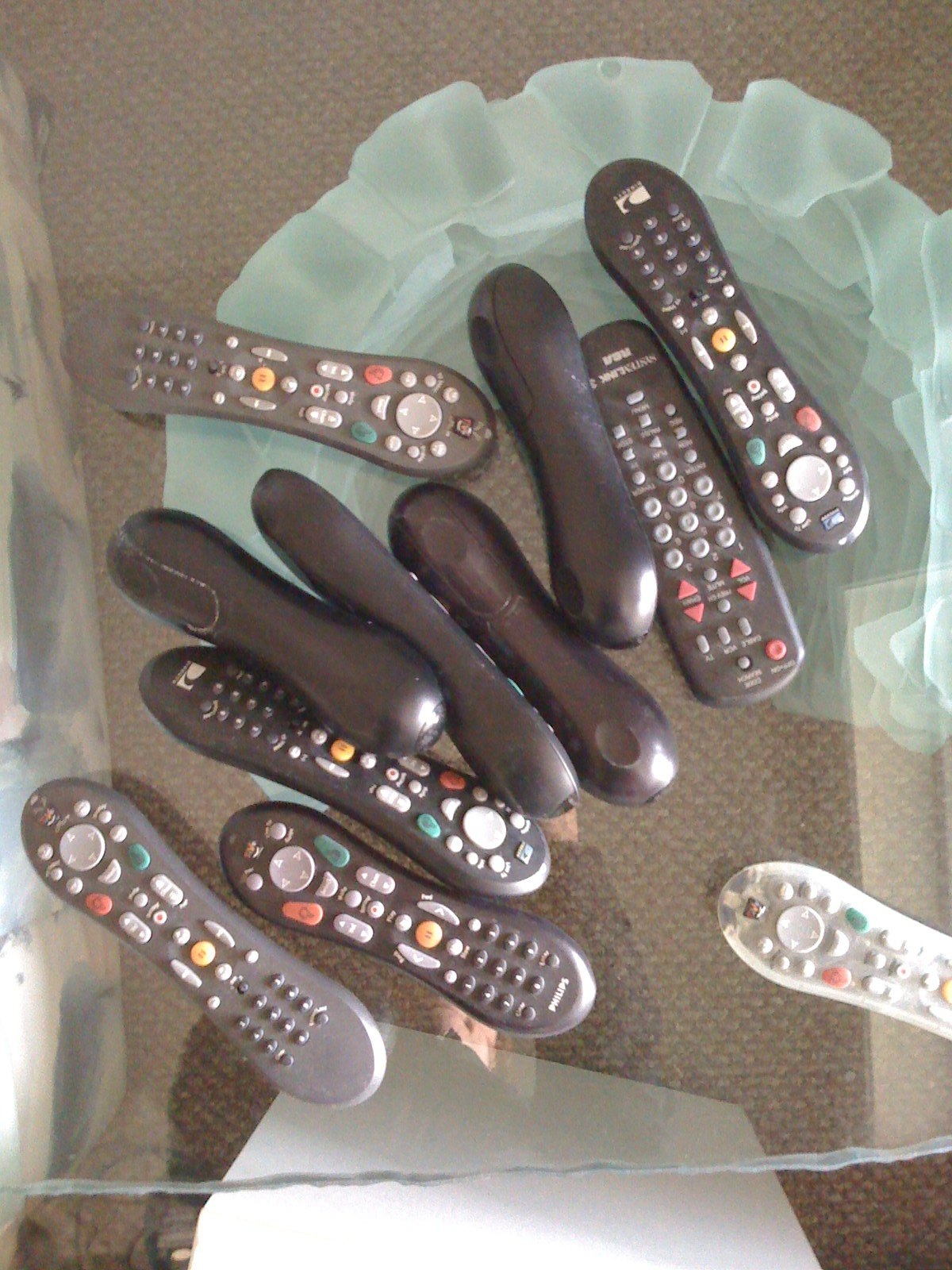This overhead photographic image captures a clear glass tabletop with a brown Berber carpet visible beneath it. The table is scattered with eleven television remote controls, predominantly black, featuring red, white, green, and yellow buttons. Most remotes have a distinct shape with a thinner center than the ends. Notably, one remote in the lower right corner appears translucent, adding an element of peculiarity. There’s a light blue, lacy-looking object in the top right corner and a white piece of fabric underneath the table. The variety in positioning of the remotes, with some showing soft-touch buttons and circular dials while others are upside down, contributes to the scattered and random appearance of the assortment.